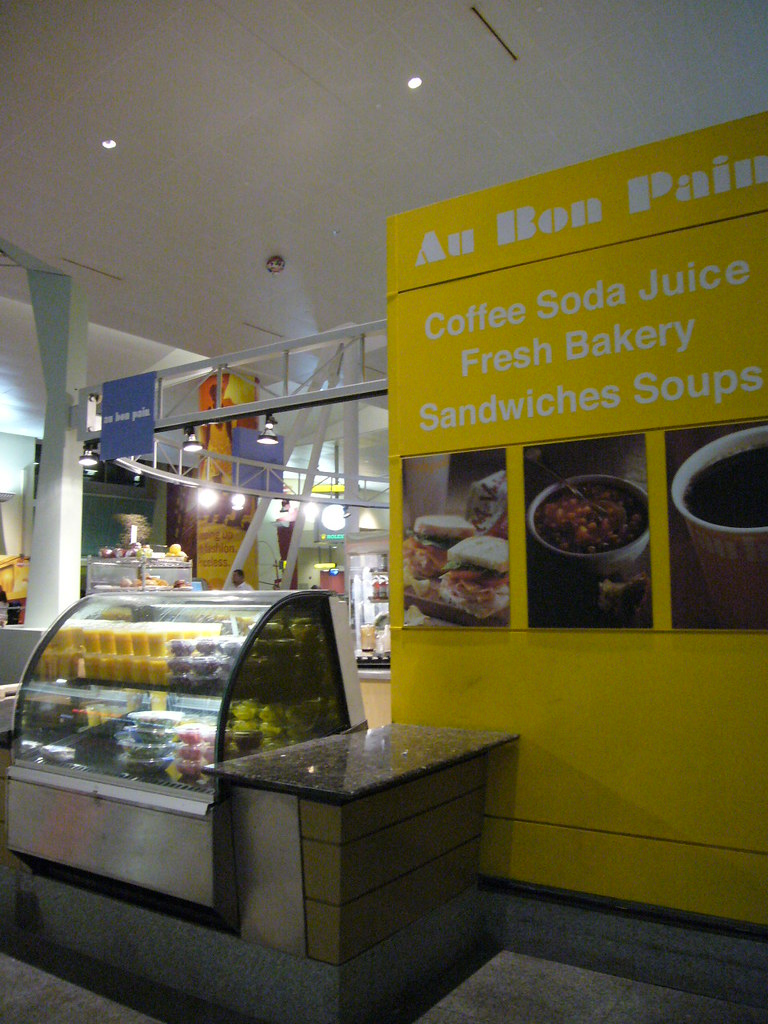The image depicts the interior of a sandwich shop or deli, prominently featuring a large yellow wall on the right side with the text "Au Bon Pain, Coffee, Soda, Juice, Fresh Bakery, Sandwiches, Soups" in white letters. Three large posters adorn the wall, displaying images of a sandwich, a bowl of soup, and a cup of coffee. To the left of the image, there's a marble counter and a refrigerated display case containing neatly arranged orange juice, various drinks, cookies, salads, and packaged fruits in yellow, red, and black plastic containers. The deli counter allows patrons to view and select items, which employees can serve. Behind the main counter area to the left, there's a clear view of the kitchen and another refrigerator. The ceiling showcases horizontal steel bars with attached lights, suggesting a layout typically found in mall food courts. The establishment appears empty, as there are no customers or staff visible, giving it a slightly closed or unoccupied atmosphere.